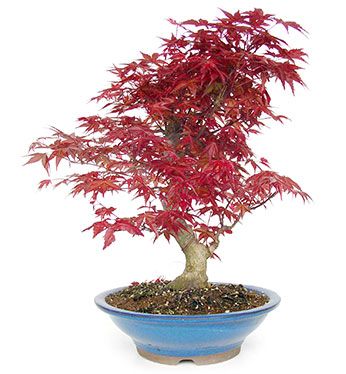The photo depicts a miniature bonsai tree with a light tan trunk and lush, delicate leaves that are a striking cherry-red to burgundy color. The tree is potted in a small, pale blue ceramic or pottery saucer with a distinctive white streak just above its grayish bottom rim. The bonsai's vibrant foliage covers its branches densely, contrasting beautifully with the brown soil in which it is planted. The tree's overall appearance is reminiscent of both an oak with its sturdy bark and the vibrant hues of a maple. Its intricate and compact form captures the essence of a miniature, well-cultivated tree.